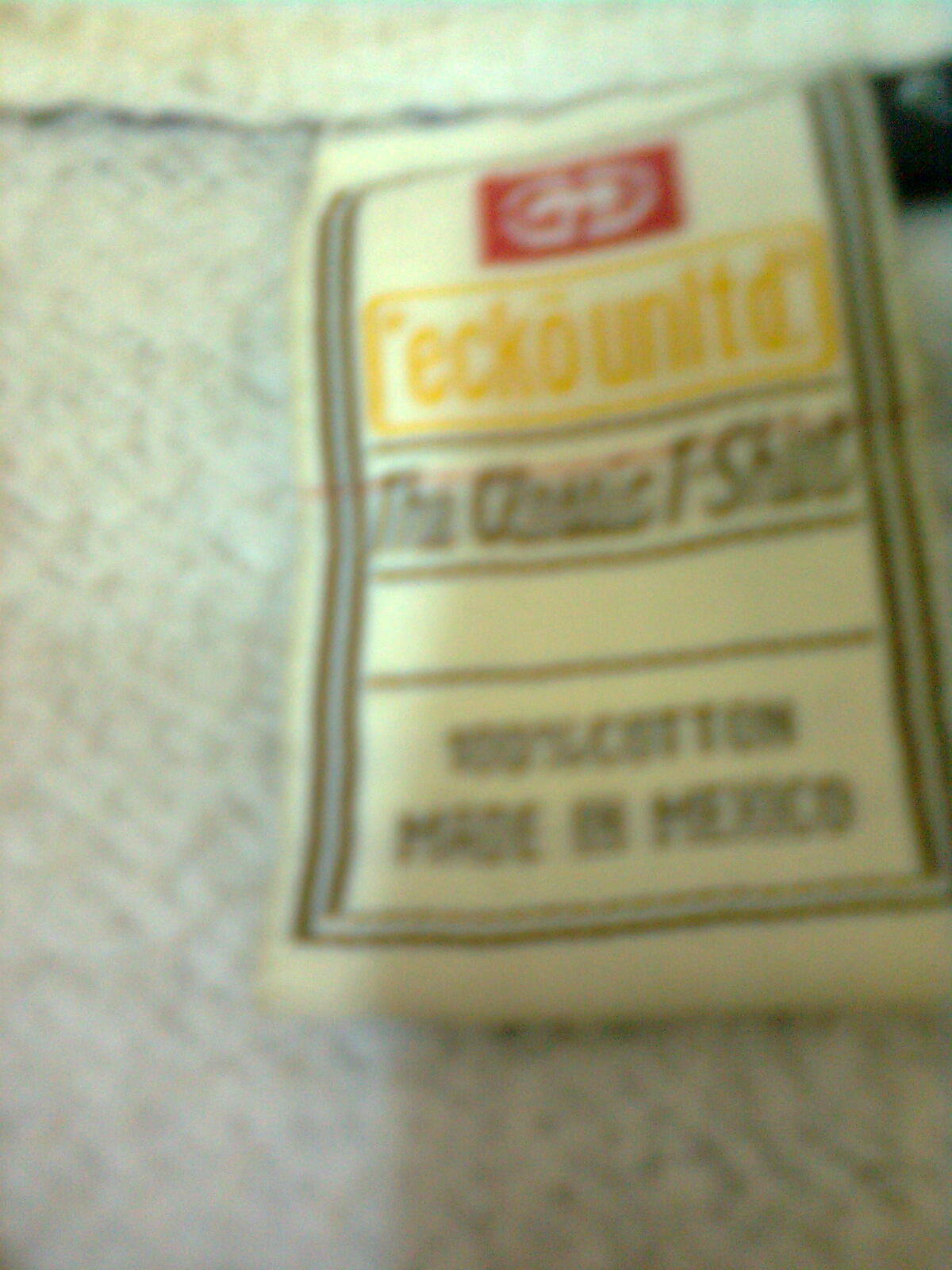The image is a large, portrait-oriented, and extremely blurry photo of a clothing label, placed beneath the collar of what appears to be a pale blue or cream beige shirt, possibly a gray t-shirt. The white tag features distinct black lines down the sides and is divided into several sections. At the top of the tag, there is a red box with white writing that is difficult to decipher. Directly below it, there is a yellow box that seems to read "RECO unit D" or "ECHO unit D," though the exact wording is unclear. Further down, surrounded by a black box resembling a frame, is black text that possibly includes the phrases "classic t-shirt," "100% cotton," and "made in Mexico."